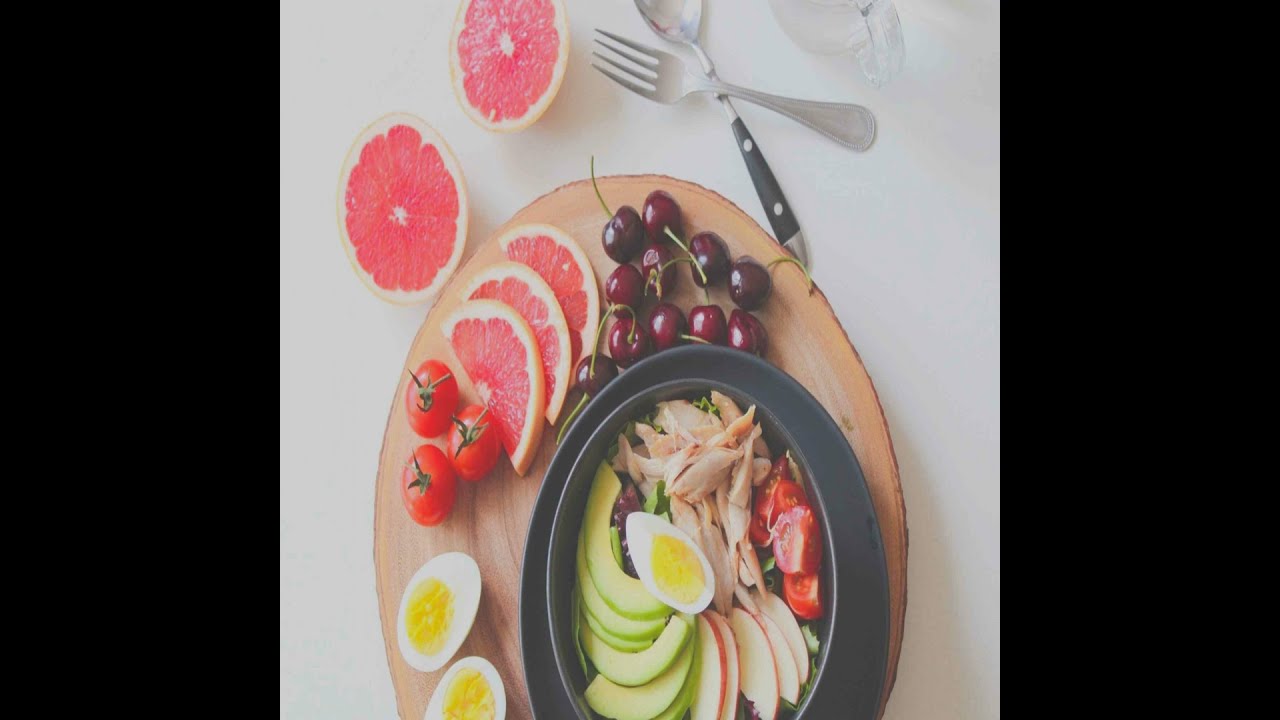The image captures an overhead view of a photogenically arranged meal set on a wooden-colored tray, bordered by thick black strips on the left and right. The picture is oriented sideways, with the plate of food centered and extending off the image's bottom edge. At the heart of the arrangement is a round bowl containing a mix of avocado, hard-boiled egg (cut in half), possibly chicken, lettuce, and some red fruits like strawberries. Positioned left of the bowl are two more sliced hard-boiled eggs, and to the right are three small tomatoes alongside three grapefruit wedges. Adjacent to these items are roughly ten cherries, contributing to the vibrant assortment. Further above in the image, a fork and spoon with a black handle cross each other, and a halved grapefruit sits to their left. The scene is completed with the edge of a glass visible at the upper portion, emphasizing the careful, artistic presentation of the meal.